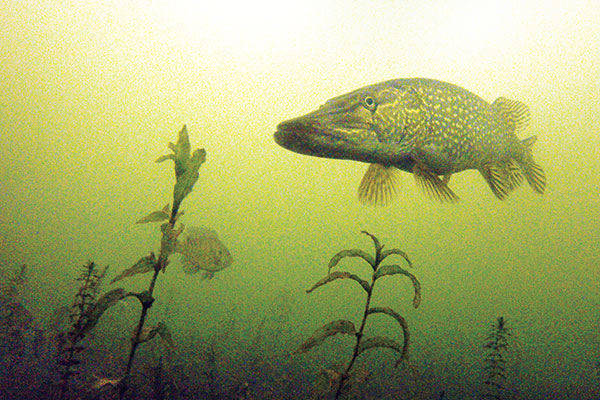This detailed underwater scene, possibly a photograph or very realistic drawing, appears to take place in a calm, murky pond, judging by the static nature of the aquatic plants and the pond-like water. Dominating the foreground is a large fish resembling a largemouth bass, characterized by a dark body embellished with sparkly dots, numerous fins, and a prominent elongated mouth area. The fish's eyes appear lethargic, giving it a somewhat laid-back expression. Further back, partially obscured by the murkiness of the yellowish-green water, are smaller fish, including one with noticeable stripes and a big dorsal fin, possibly a perch or sunfish. Bright sunlight penetrates the water, illuminating the scene from above and casting a lighter yellow hue near the top, contrasting with the lime-green tint prevalent at greater depths. Lush, vibrant aquatic plants with green leaves spread from the bottom of the image, adding texture and depth to this serene underwater tableau.